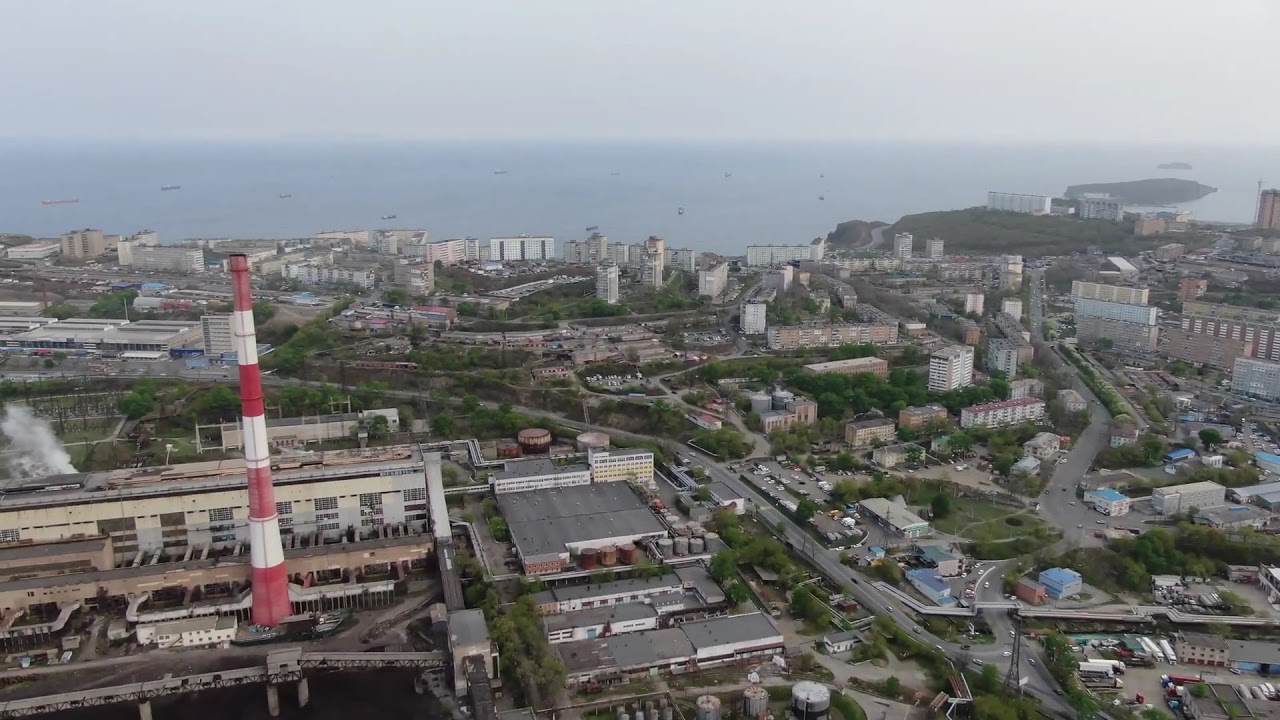The color photograph, taken from a high vantage point, offers a vibrant, clear, and detailed aerial view of a bustling coastal city during the daytime. The image, captured in landscape orientation, spans a broad urban expanse with a dense network of buildings and roads teeming with traffic. The bottom two-thirds of the photo prominently features intricate roadways filled with cars and reveals a mixture of commercial and industrial zones, particularly noticeable in the lower left corner. Here, a striking red and white horizontally striped tower stands out amidst the surrounding structures, rising approximately 50 feet with a narrow, candy-cane-like appearance. Billowing smoke or exhaust is visible from a building behind the tower, contributing to the industrial scene. The upper third of the image is dominated by a large body of water, extending horizontally and meeting a light gray sky at the very top. The natural light of the daytime setting enhances the vibrancy of the city's range of colors, from the grays and whites of the buildings to the greens of urban vegetation, providing a vivid, realistic representation of the coastal metropolis.